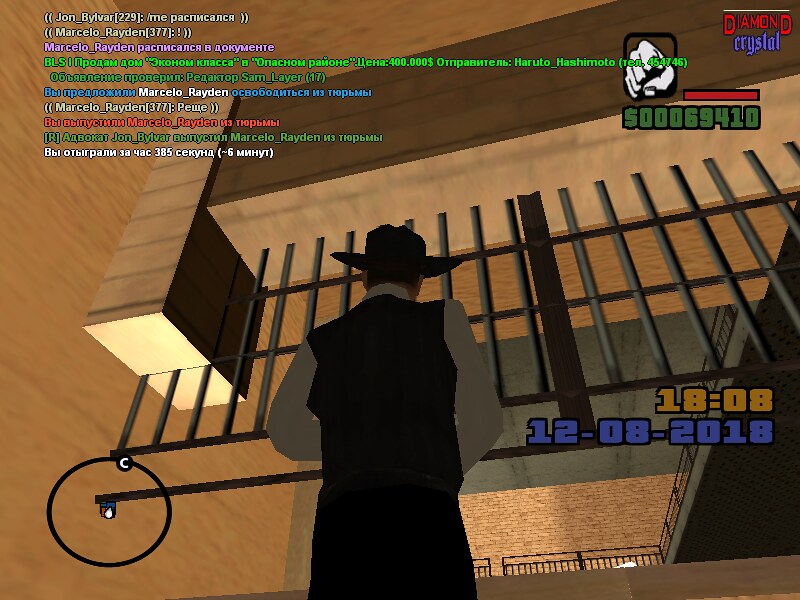### Detailed Descriptive Caption

In the screenshot of a video game, a man stands inside a high-rise building, appearing to look up towards an indoor balcony above him. He is dressed in a black vest over a white-collared shirt, black pants, and a black cowboy hat. At the top of the image, the text reads "Diamond Crystal Diamond" in various colors—red, blue, and perhaps indicating the game's title. In the upper right corner, a chatbox is visible with text in another language. The chat includes messages like "john bauver bylvar 229" and "me pancasara pacnmacana," enclosed in double parentheses. The timestamp on the chat reads "18:08," and the date displayed on the image is "12-08-2018."